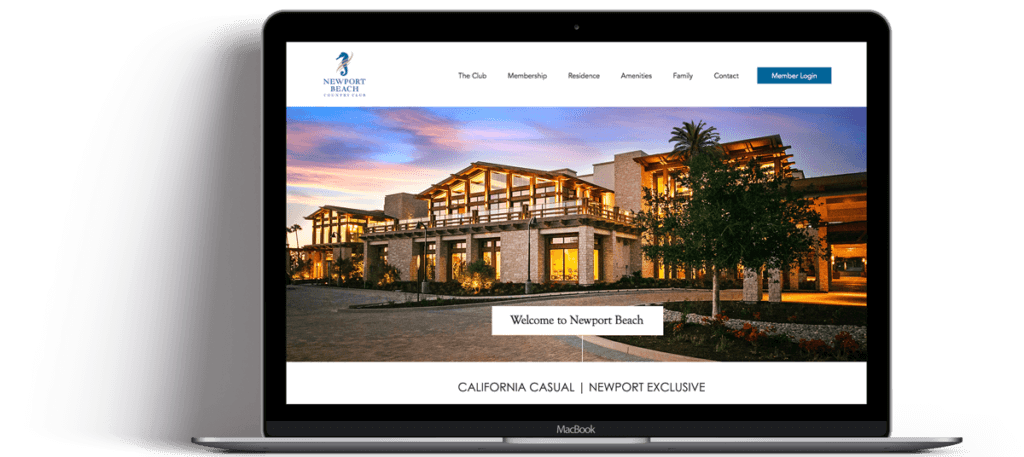### Descriptive Caption:

The image showcases a sleek MacBook laptop displaying the Newport Beach Country Club's website. Prominently featured on the screen is the club's elegant seahorse logo against a clean and sophisticated layout. The website's navigation menu at the top offers easy access to essential sections, including "Club," "Membership," "Residents," "Amenities," "Family," "Contact," and a prominently highlighted "Member Login" button in blue, designed for user convenience. Below the navigation, a stunning panoramic photograph captures the country club bathed in the warm hues of sunset, with pink and blue clouds adorning the sky and the club's building warmly illuminated, exuding a welcoming atmosphere. Superimposed on this captivating scene is a button labeled "Welcome to Newport Beach," followed by the text "California Casual, Newport Exclusive," encapsulating the club's unique blend of relaxed luxury. This image represents the enticing homepage geared towards both potential and existing members of the Newport Beach Country Club.